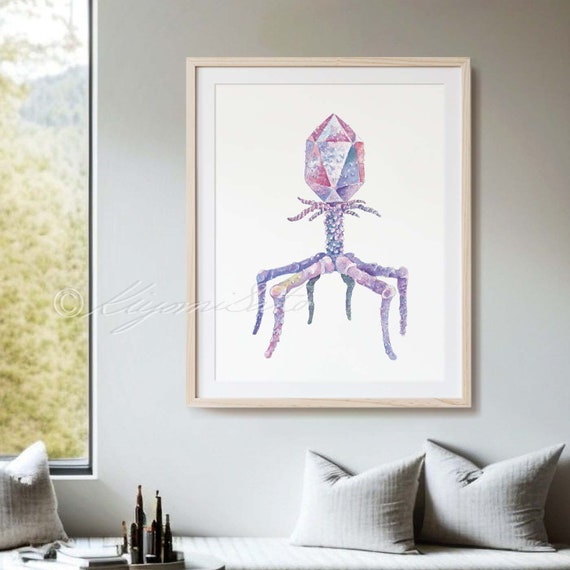This photograph captures a serene interior setting dominated by a gray-white wall. Central to the wall is an eye-catching piece of art encased in a beige frame with a white mat. The artwork, featuring a white background and rendered in soft pastel hues of blue, red, lilac, and yellow, depicts an abstract figure reminiscent of a creature with six articulated legs extending from a singular vertical pole post. The figure's upper section features tendrils and a geometric head that resembles a geodesic dome. To the left of this central piece, just a small part of another painting is visible at the bottom right corner, though not enough is shown to identify its content.

Below the artwork, there is a seating area that might be a bed, bench, or couch, adorned with three gray pillows that appear indented at the top, suggesting recent use. To the lower left on this surface, a dark gray sculpture or statue adds a touch of elegance. A tray with small dark bottles also sits atop this area, contributing to the minimalistic decor. On the far left edge of the photo, a portion of a window reveals a glimpse of outdoor greenery and sky, introducing a hint of natural light into the scene. The muted pastel tones of the entire setting provide a calm and inviting atmosphere.